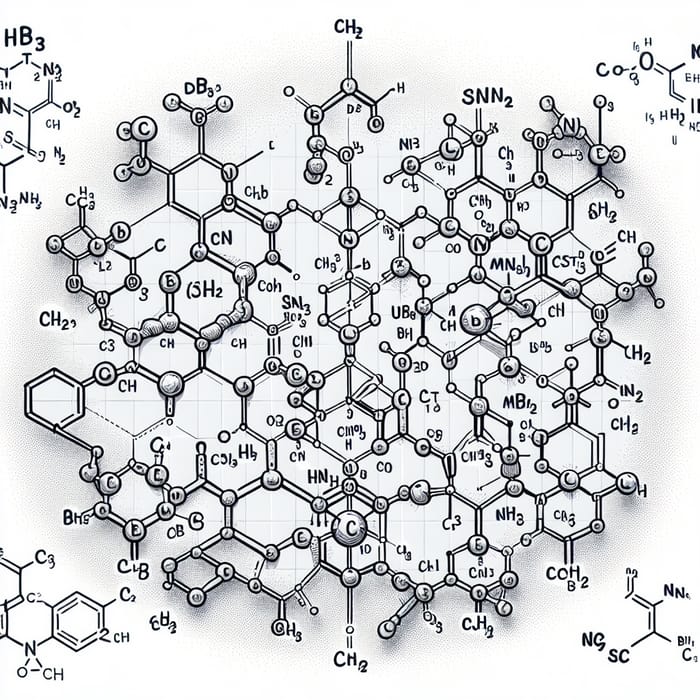This black-and-white image appears to be a complex scientific diagram, likely hand-drawn on graph paper, depicting the Lewis structure of various covalent compounds. The central focus is a hexagonal molecular structure with multiple lines and atoms interconnected, resembling a detailed chemical chart from a textbook. Key chemical symbols and formulas, such as CH2, SNN2, CO2, and others like HB3, DB3, and 10H, are dispersed throughout the diagram, though not in a recognizable pattern. This intricate image includes numerous elements, with notable features such as a large carbon chain at the bottom and several smaller structures, possibly alkanes or alcohols, unconnected on the left and right sides. The chart lacks explanatory text, leaving its exact purpose or identity ambiguous.